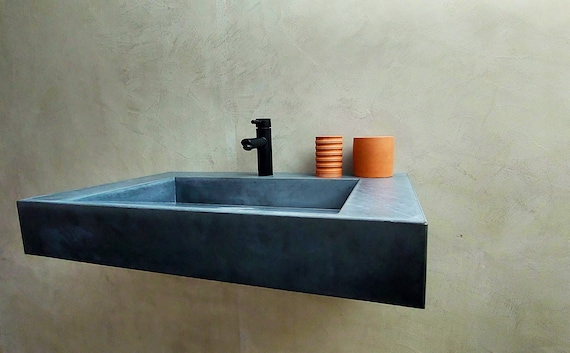The photograph appears to be a computer-generated image of a modern, floating sink attached to a wall with no visible drainage pipes. The sink is rectangular and primarily light blue with darker shading along the sides. The wall behind the sink is a spackled light brown with a hint of bluish hue. Centered toward the bottom and slightly to the left, the sink features an opening in the center for water drainage. A sleek black faucet, possibly made of plastic or metal, is installed above the sink. To the right of the faucet are two clay-colored containers: one is ridged and the other is longer and smoother. The overall setting suggests an indoor environment, likely a bathroom, characterized by a cement-like wall and minimalistic design.